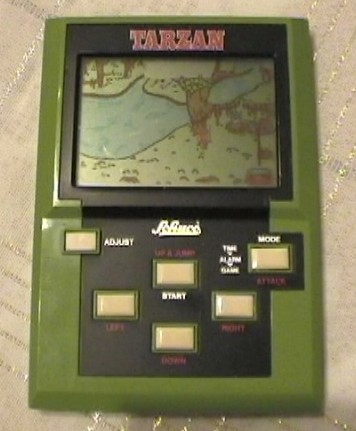This photo displays a vintage handheld video game, seemingly from the 1980s, housed in a navy green case. Prominently, the title "T-A-R-Z-A-N" is emblazoned in red letters at the top of the device. Below the title is a small, calculator-like screen depicting a grassy terrain with rocks, trees, and a pond or stream, suggesting a natural setting conducive to animal life. The foreground features more trees and rocky patches, adding depth to the game environment.

At the bottom of the screen, there is a series of yellow rectangle buttons, each labeled for specific functions: "Start," "Adjust," "Mode," "Left," "Right," and "Attack." Some of these buttons have additional text beneath them, in red, which is unfortunately too blurry to decipher. The black interior frame of the screen contrasts sharply with the overall green casing of the handheld device. The entire gadget appears to be around eight to ten inches tall and is photographed against a beige cloth backdrop with visible stitching, suggesting a casual home setting, possibly for an online sale listing.